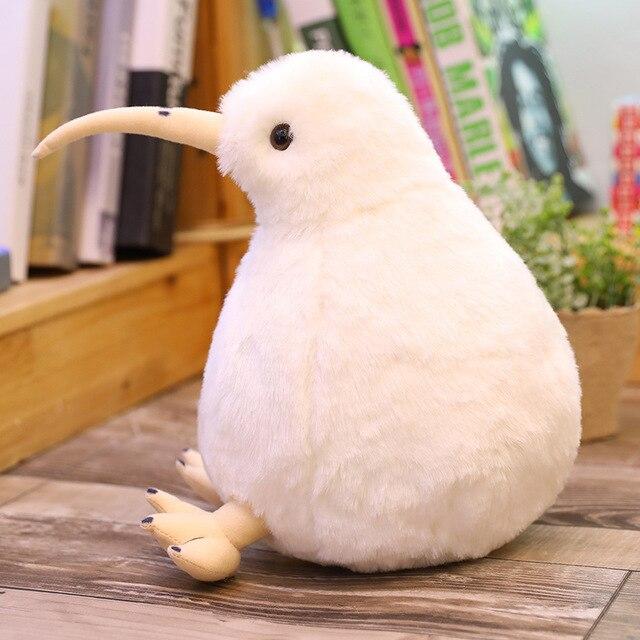The image captures an adorable stuffed kiwi bird sitting on a wooden floor. The bird is characterized by its white, fluffy, oval-shaped body, a roundish head, and a long, yellowish, carrot-like beak with a soft, muted color. The kiwi's little legs are propped up with three toes on each foot, featuring small black dots. Behind the kiwi, a wooden bookshelf is visible, holding several books. One of the books showcases Bob Marley's face on its cover, while the other titles are blurred but display a variety of colors including black, white, tan, lime green, and plum. Additionally, a small potted plant with orange and white hues adds to the cozy, detailed scene.